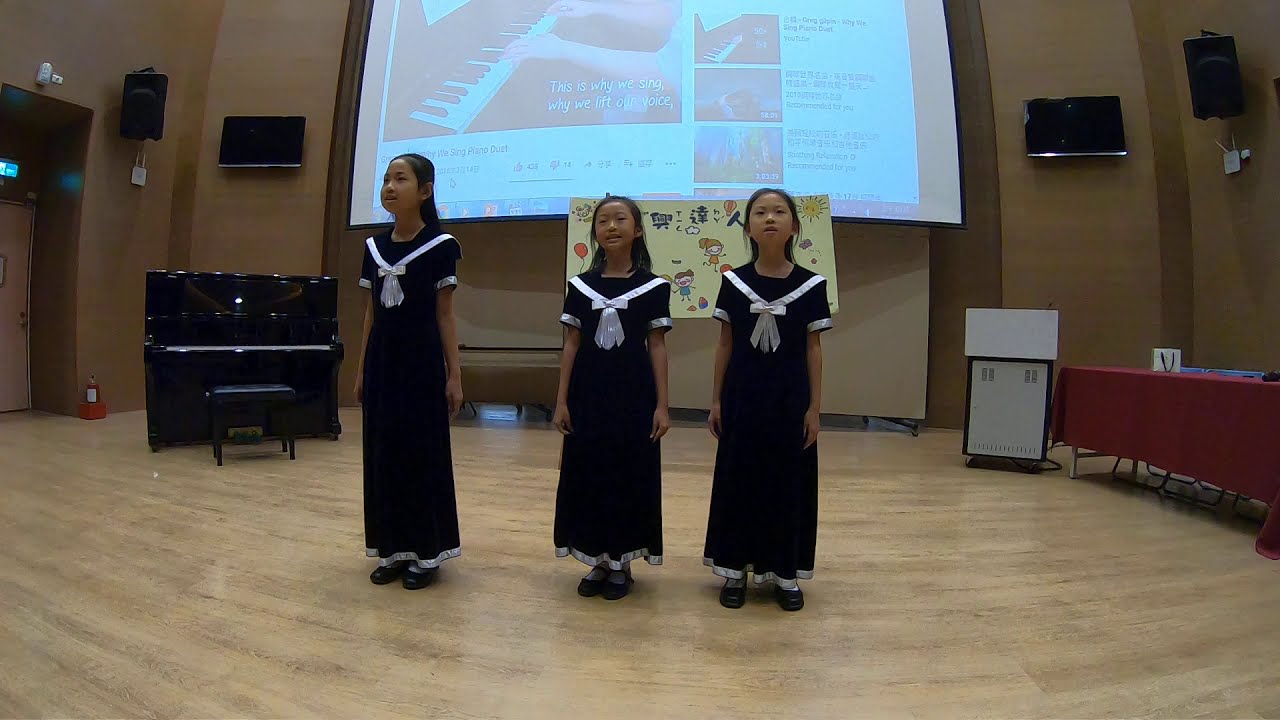The photograph captures three young Asian girls, approximately 9 or 10 years old, performing indoors. They are standing on a glossy, light brown wooden floor in a large room, likely designated for performances or classroom activities. The girls, each with long dark hair, are dressed in distinctive, floor-length black dresses with white ribbons tied over their shoulders, resembling sailor dresses. Their arms rest by their sides as they face forward, with the exception of the girl on the left, who is turned slightly diagonally.

The top portion of the image reveals a tan-colored wall featuring two small black TV screens on either side of a large white screen. This central screen displays a projected YouTube video showing someone playing the piano. Directly beneath the screen appears to be a poster adorned with various icons and pictures. To the left of the girls stands a black upright piano and a doorway, while to the right, there's a long table covered with a red tablecloth and a whiteboard beside it. Additionally, the walls are equipped with multiple speakers: two square and two rectangular, positioned symmetrically around the large screen.